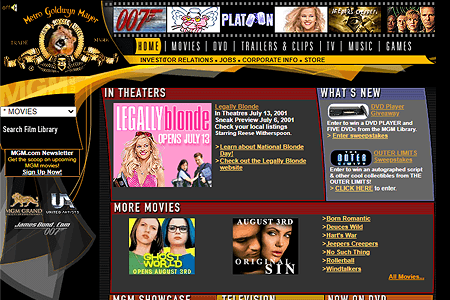The image features a prominently placed yellow Metro-Goldwyn-Mayer (MGM) logo with their iconic lion at the top-left corner. Above this logo, the text "007" and "Platoon" are displayed, alongside a promotional image from the movie "Legally Blonde." Below, in white text, it reads: "Home, DVDs, Trailers and Clips, TV, Music, Sales."

Further down, the image advertises the theatrical release of "Legally Blonde," slated for July 13th, 2005, with a sneak preview on July 4th, 2001. It encourages viewers to check their local listings and highlights Reese Witherspoon as the star. Additionally, it mentions National Blonde Day and invites users to visit the "Legally Blonde" website for more information.

The image also includes a section labeled "What's New," promoting a DVD player giveaway and an "Outer Limits" sweepstakes. Under the "More Movies" segment, there's information about upcoming releases: "Ghost World" on August 23rd, "Original Sin" on August 3rd, and other genres and titles like "Romantic," "Wild," "War," "Jeepers Creepers," "No Such Thing," "Rollerball," and "Wind Bullets."

Finally, a search bar is positioned on the left side of the image, facilitating easier navigation for users.